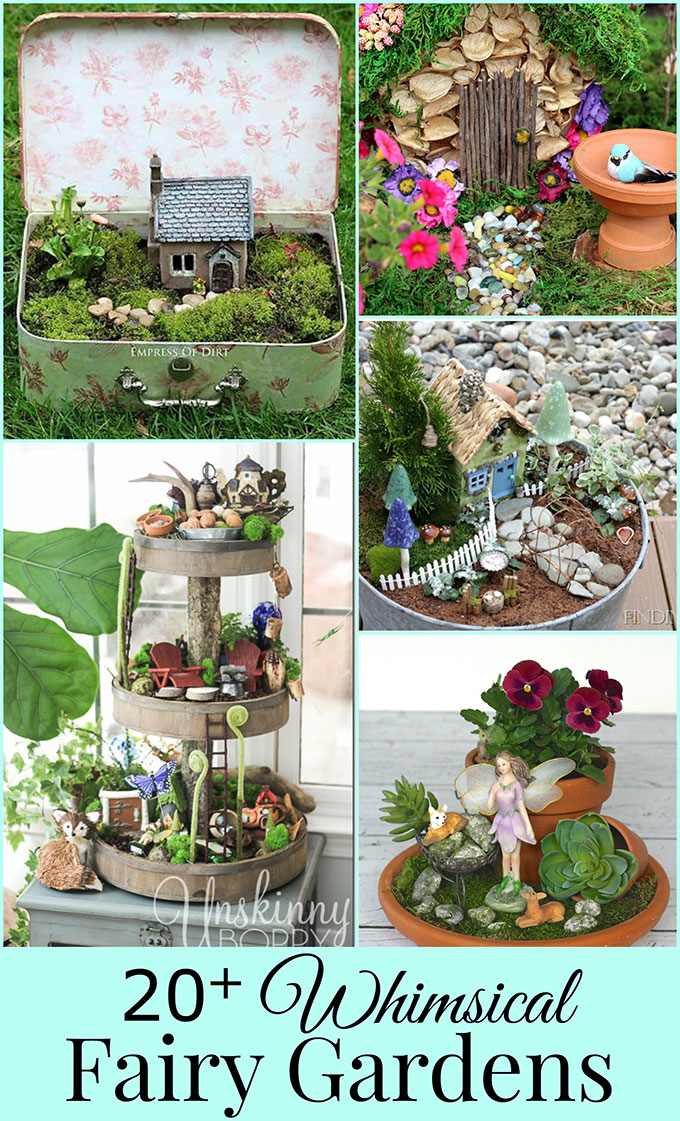This image is the cover of a digital e-book titled "20 Plus Whimsical Fairy Gardens," prominently displayed against a light bluish-green background with black text. The cover features a collage of five distinct, intricately designed fairy garden photographs. On the left side, the upper image showcases a fairy garden ingeniously created inside an old metal lunchbox. This garden includes a tiny house, miniature stone walkways, delicate flowers, and a petite figure with the inscription "Empress of Dirt." Below it, a whimsical three-tier fairy garden made from what looks like a dessert stand or birdbath is adorned with various magical plants, tiny red wooden chairs, and ladders connecting the levels. On the right side, the top image presents an outdoor fairy garden built into a hillside with a stone and wood stick door and a colorful stone pathway. Beneath it, another garden is housed in a large metal bucket, featuring a small greenhouse with a hay-like roofing, trees, fencing, and mushrooms. The bottom right image showcases a fairy garden in a terracotta pot saucer, centered around an actual fairy statue surrounded by flowers. Each garden creates a captivating miniature fairy world, emphasizing the enchanting and creative aspects of this e-book.